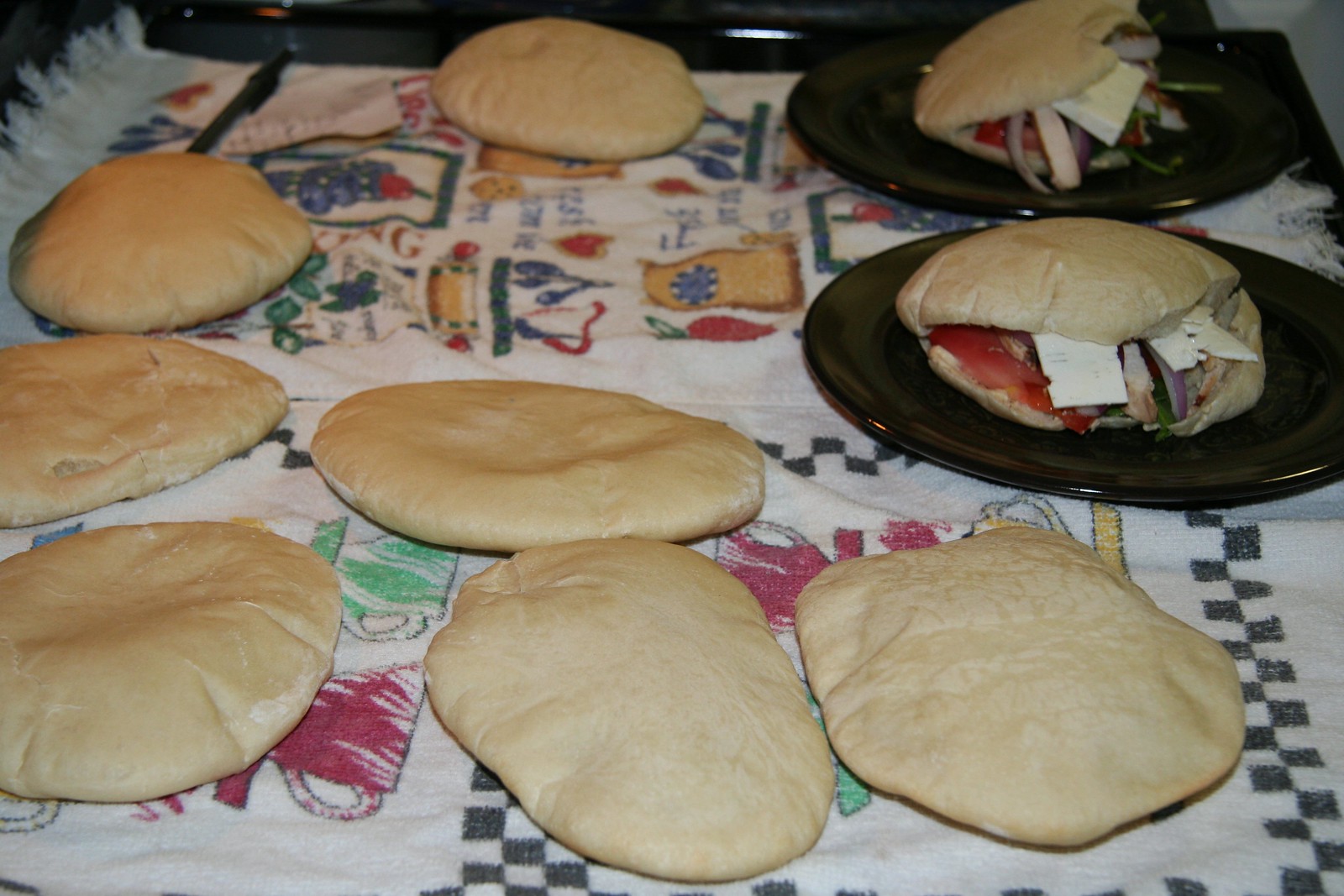This image displays a close-up of nine freshly baked pita breads on colorful kitchen towels adorned with various patterns of teacups, fruits, and baking symbols. Seven plain pitas are neatly arranged on the towels, while two stuffed pitas, filled with cheese, feta, chicken, purple onion, lettuce, and tomato, rest on black plates. The arrangement suggests a mixture of preparation and presentation, capturing the freshness and anticipation of a delicious meal.